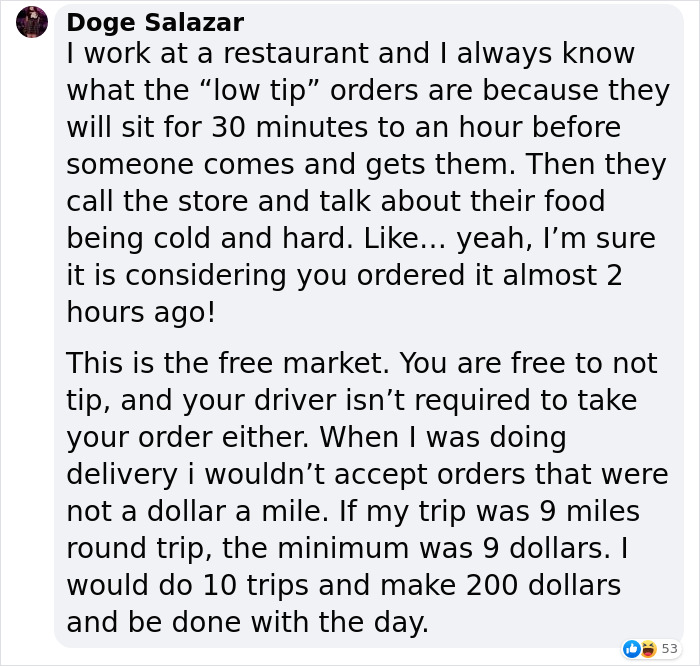This is a screenshot of a message from Dodge Salazar, encapsulated in a thin gray border. The message itself is presented within a gray box, written in black text. Adjacent to the message is a small circular icon featuring Dodge’s profile picture. Dodge's message highlights his experience working at a restaurant, stating: "I work at a restaurant and I always know what the low tip orders are because they will sit for 30 minutes to an hour before someone comes and gets them. Then they call the store and talk about their food being cold and hard. Like yeah, I’m sure it was considering you ordered it almost two hours ago. This is the free market. You are free to not tip and your driver isn’t required to take your order either. When I was doing delivery, I wouldn’t accept orders that were not a dollar a mile. If my trip was nine miles, round trip, the minimum was $9, I would do 10 trips and make $200 and be done for the day." Below the message, there is a Facebook-like emoticon indicating the message received engagement, accompanied by a laughing emoji and the number 53, suggesting it has garnered 53 laughs or reactions.